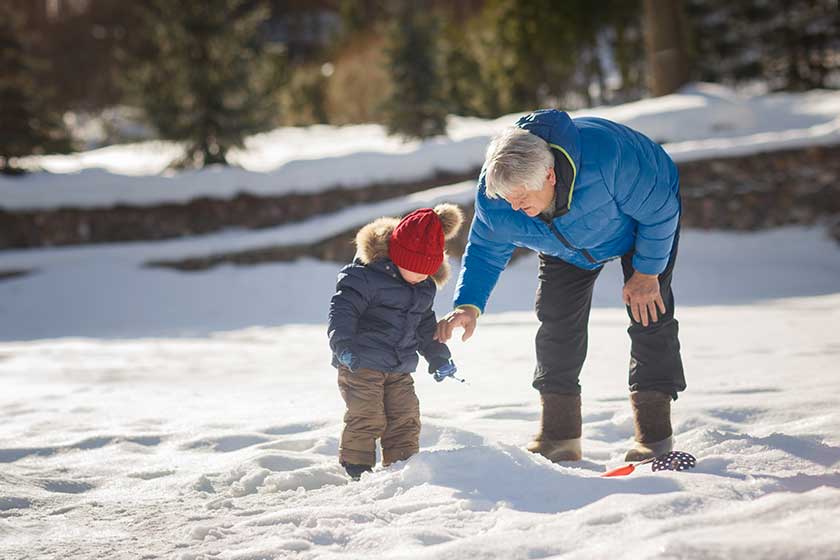In this captivating winter photograph, an elderly man with gray hair, dressed in a sky blue down coat and khaki pants with boots, is bending over with his right hand extended towards a toddler. The toddler, clad in a dark blue down coat with a tan fur hood, tan pants, and a red hat adorned with a fur pom-pom, appears to be holding something in his mittened hand. The pair seems to be focused on an object in the snow between them: a black circular disc with red dots, a red shovel, and an orange item resembling a feather or toy. Behind them, the snow-laden ground is dotted with numerous footprints, leading up to a dark stone wall also covered in snow. Above the wall, at the extreme rear of the photo, a mix of dark brown and light brown trees forms a wintery backdrop with a touch of evergreen, adding to the seasonal atmosphere.